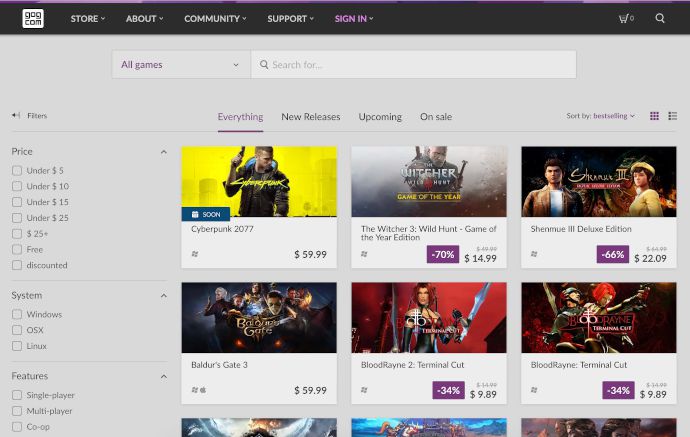The image is a horizontally rectangular screenshot from a website. In the upper left corner, the GOG.com logo is prominently displayed. Adjacent to the logo, moving from left to right across a black horizontal banner, are navigation options labeled Store, About, Community, Support, and Sign-In, each with a drop-down arrow for additional selections. On the far right of the banner, icons for the Shopping Cart and Search functions are clearly visible.

Below the banner, the main content area has a light to medium gray background and is centered within the frame. A search field is placed prominently at the top. On the left side of the screen, a vertical pane contains various filter options. These filters are categorized by price ranges (Under $5, Under $10, Under $15, Under $25, and $25+), alongside options for Free and Discounted items. Below the price filters, system compatibility options are listed, including Windows, OS X, and Linux. Further down, there are filter options for game features such as Single Player, Multiplayer, and Co-op.

To the right of the filters, a horizontal line of options allows the user to select viewing categories: Everything, New Releases, Upcoming, and On Sale. Below these categories, six images of different games are displayed, each accompanied by pricing information.